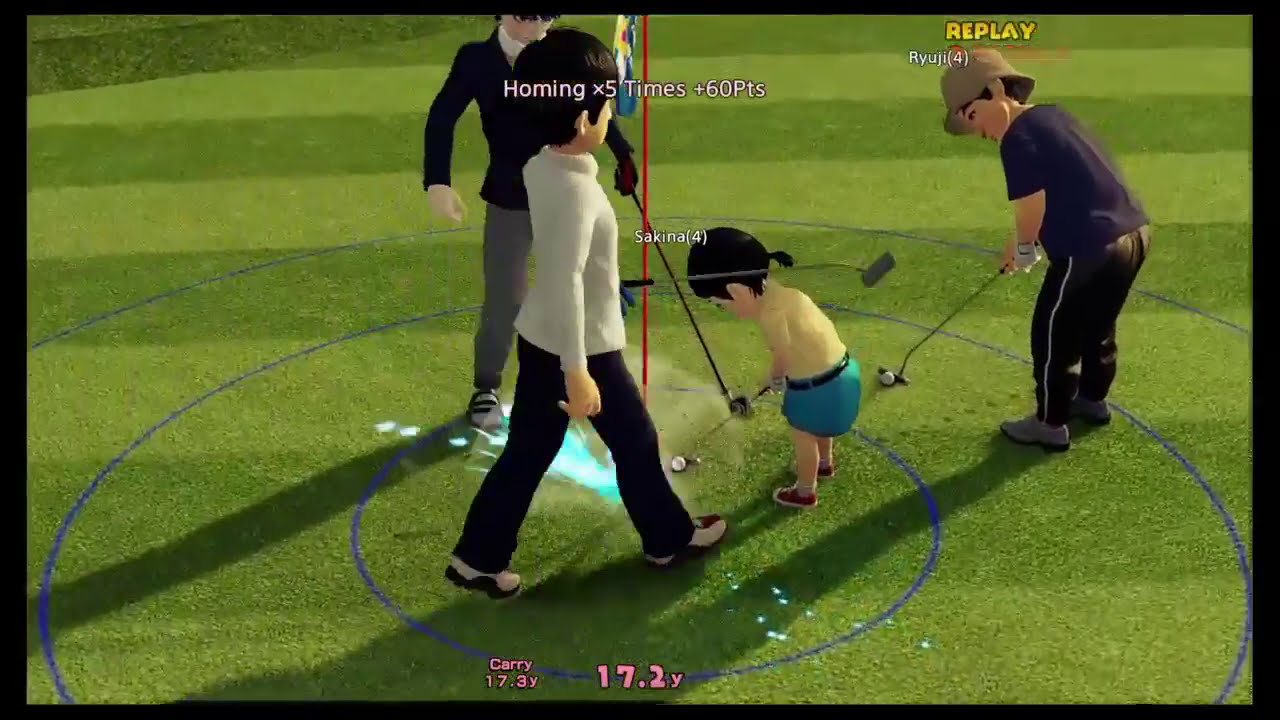The image depicts a digital game scene featuring four characters on a golf course, all involved in putting. On the far right is a male golfer, hunched over with a golf club in hand, preparing to putt. He wears a blue shirt, black pants with a white stripe, gray shoes, a brown hat, and has brown skin with black hair. Above him, the text “Replay” in yellow, alongside the name "Ryuzi" and the number four, identifies him in the game. 

Next to him on the left is a young child with black hair tied in a ponytail, dressed in a yellow shirt, teal shorts, and red shoes, also holding a golf club aimed at a ball. 

To the left of the child stands an adult with a light-colored long-sleeve turtleneck, black pants, white and red shoes, and short black hair, depicted walking towards the child. 

Behind this person, another adult is observed wearing a dark long-sleeve jacket, gray pants, and holding a golf club pointing downwards. This individual has a white ring around their neck.

Central text on the screen reads "Homing x5 +60 points," along with “Sykirna 4” and "Carry 7.3 V, 17.2 Y" indicating game statistics. A red line runs vertically in the center with a light teal glow extending to the upper left. The ground beneath the characters features concentric blue circles, expanding outwards, adding dynamic visual effects to the gaming environment.